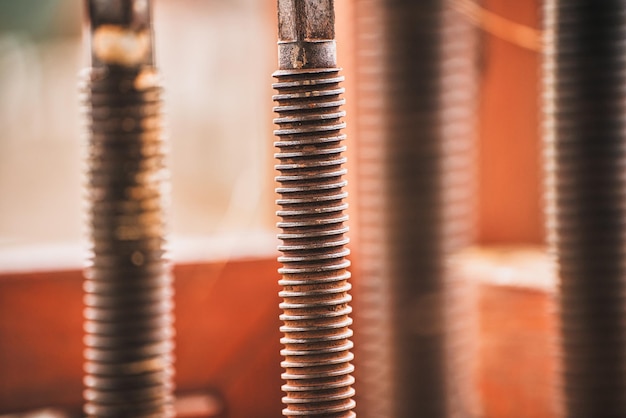This photo features a set of four aged, rusted, threaded metal bolts, all standing upright. The bolts, with their square nubs at the top showing distinct signs of wear and tear and initially silver surfaces now marred by rust and brown discoloration, dominate the image. The threads, appearing as uniformly spaced rings spiraling down each bolt, are clearly visible. A closer look reveals one bolt in sharp focus in the foreground, while the remaining bolts in the background appear slightly larger but blurry. Variations in size and positioning across the image add depth, with the bolts placed from left to right across the frame. The scene includes subtle hues of orange, yellow, green, silver, and gray, and the overall setting against a blurred background that resembles an industrial area with a partially visible white and red wall. Additionally, there is a hint of a rope or wire dangling in the top right corner of the image.